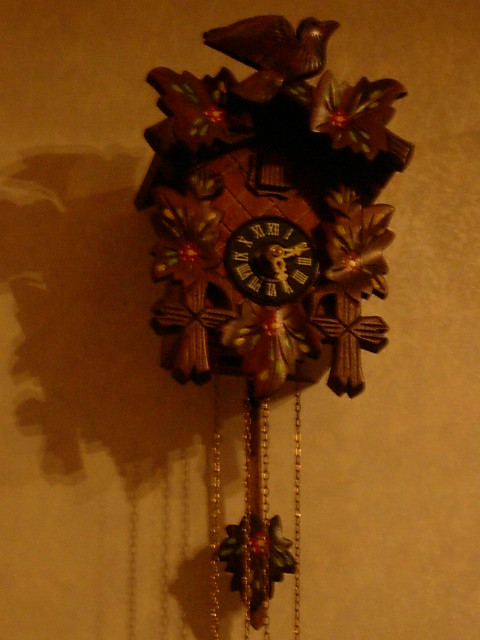This image captures a slightly blurry and grainy photograph of an elaborate cuckoo clock, meticulously crafted from dark wood. The clock is mounted on a dark yellowish-brown wall, and its intricate design stands out despite the image quality. At the heart of the clock is a small, centrally positioned, albeit slightly lower part, time-telling dial. This dial is black with Roman numerals, featuring ornate white hour and minute hands. The clock's face is framed within a larger wooden structure adorned with detailed carvings. Surrounding the dial, the woodwork includes two crosses and multiple leaf-like shapes, artistically resembling foliage. Prominent at the very top is a bird with outstretched wings, appearing poised for flight. Contributing to the clock's functionality and charm, four gold chains and a wooden pendulum—designed like a leaf with green leaf accents at the end—dangle below, completing this intricate timepiece.